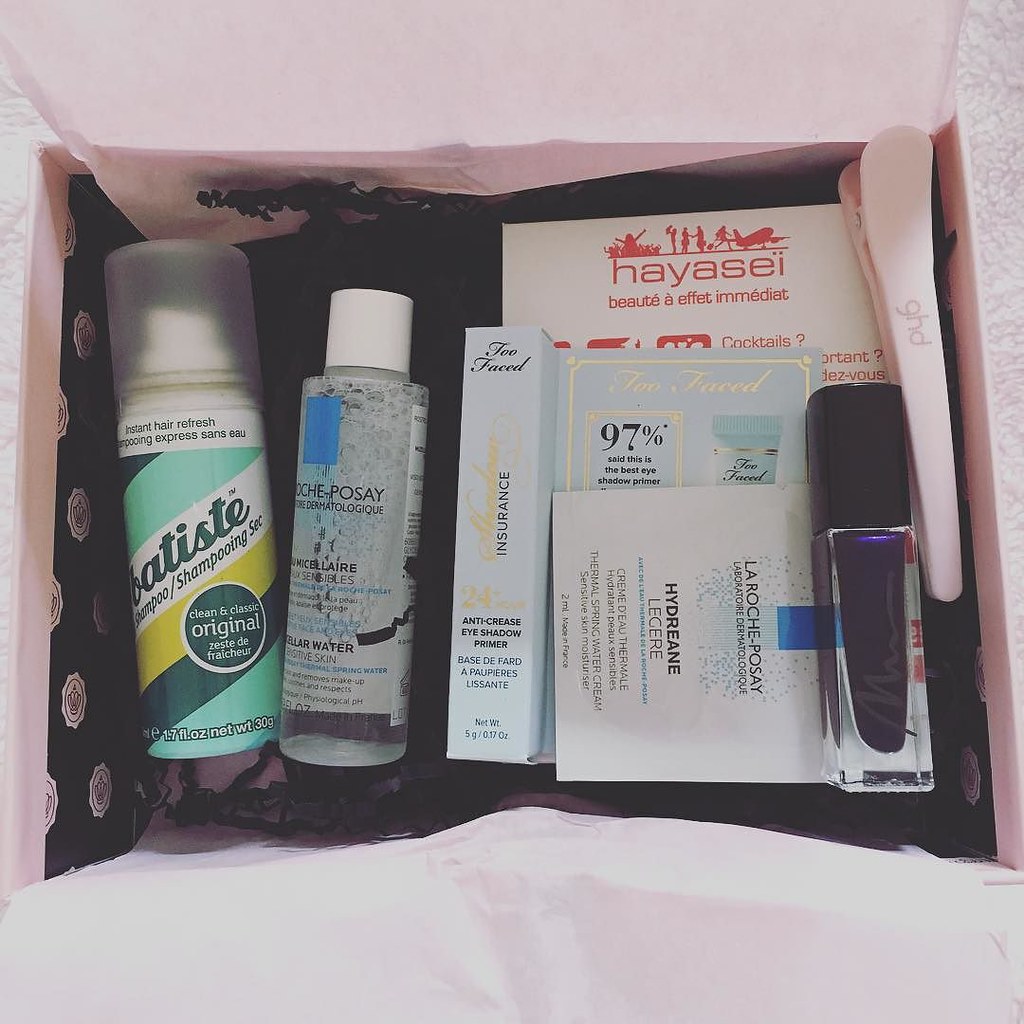The image showcases a neatly arranged collection of beauty and skincare products against a decorative background. The top and bottom areas of the backdrop are light pink, accompanied by a detailed pattern on the left and right edges, resembling a tiled floor with gray squiggly lines. 

At the center of the composition is a black background adorned with silver or white medallion motifs on the sides. Prominently featured within this black box is a container labeled "Hair Refresh," designed with dark green, light green, white, and yellow horizontal stripes. The label includes a circular emblem stating "Clean and Cleanse, Original."

Adjacent to this is a clear bottle with a white cap, featuring gray lettering that is somewhat difficult to discern, as well as a white label wrapping behind it. To the right, there's an eye shadow palette contained in a white box with the word "Insurance" inscribed in black.

Next to the eye shadow, two overlapping packages are displayed. The top package is white, while the one beneath it is light gray with a grayish outline and some lettering, although the text is not fully readable. Noteworthy is a phrase in black reading "97%." Behind these packages, a third white packaging sheet stands out, with bold red letters spelling "H-A-Y-A-S-E-I," followed by text in French. The package features an image of people and an airplane in the corner.

On the far right, a pink hair clip is shown, which flares out at the top and tapers at the bottom, marked with the letters "G-H-D." Below the clip, a small clear bottle with a black cap is visible, containing a dark purple liquid.

The curated arrangement and the vibrant mix of colors and textures in the image make for a visually engaging and detailed scene.